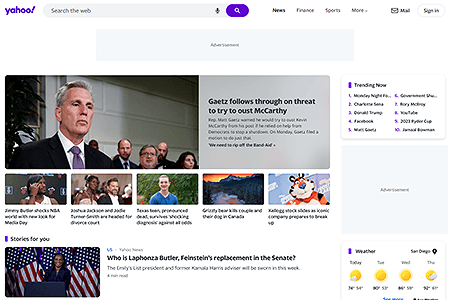The Yahoo front page is prominently displayed with various elements that are instantly recognizable. In the upper left-hand corner, the iconic Yahoo logo appears in all-purple letters with an accompanying purple exclamation point. To the logo's right is a search bar labeled "Search the web," featuring a microphone symbol for voice searches and a clickable purple button with a white magnifying glass icon.

Below the search bar are four navigational tabs labeled "News," "Friends," "Sports," and "More." Adjacent to these tabs is an envelope icon labeled "Mail" and a "Sign In" button. Beneath this navigation bar is a light gray box marked for advertisements, though currently empty.

An image headline titled "Gates Follows Through on Threat to Try to Oust McCarthy" dominates the central area. The image shows a white wall background with an audience of at least five people—three men and two women—focusing on the scene. Of these, one man is Black while the others' descriptions aren't clear.

Additional smaller images and captions follow below. One sub-image appears to show a Black man in an NBA jersey pulling his hair back. Another image potentially features a Black woman with a white man and a smiling, clean-shaven boy in a blue V-neck T-shirt. Further down, a scenic photograph depicts a beautiful sunrise or sunset over verdant pine forest hills, with a mountainous backdrop and a body of water.

To the right of this scenic image, Tony the Tiger is pictured, followed by an advertisement showcasing a woman standing in front of American flags. The accompanying text reads, "Who is LaFonza Butler, Feinstein’s replacement?" The image shows a woman of color smiling at a gray podium in front of American flags, though some additional text is hard to make out.